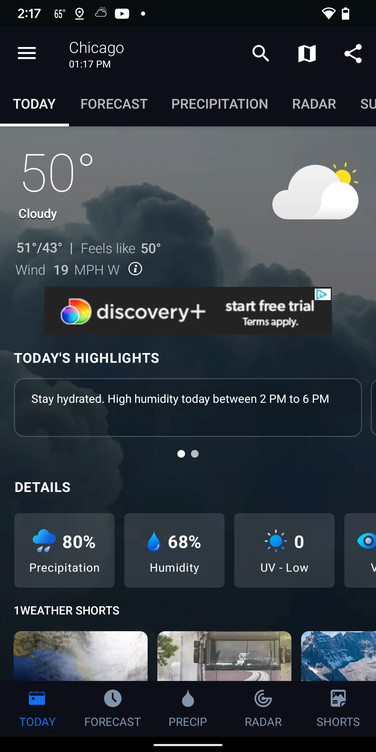Here is the cleaned-up and detailed descriptive caption for the screenshot of the weather app:

---

The screenshot captures a weather app interface, primarily focused on the current weather details and forecast. In the upper left corner, "2:17 PM" is displayed, adjacent to a "65 degrees" temperature indication. Nearby are three symbols followed by a dot and icons for Wi-Fi and battery status.

To the right of the time and temperature, "Chicago" is prominently displayed above "01:17 PM." Close to this, a search magnifying glass icon, another unidentifiable symbol, and a connected dots icon are visible. Beneath this header, in capital white letters, "TODAY" is written, followed by sections labeled "Forecast," "Precipitation," "Radar," and a partly visible section starting with "SU."

Below these sections, "50%" is indicated, with "Cloudy" beneath it. The background image is cloudy and appears to be taken at nighttime. On the right side, there is a larger icon of a cloud with the sun peeking out from behind it. Directly under "Cloudy," it states, "51° / 43°," followed by "Feels like 50°."

The subsequent details include "Wind 19 MPH W," with an informational icon next to it, followed by a rainbow icon and an advertisement for Discovery+, stating "Start free trial, terms apply." Underneath this, "TODAY'S HIGHLIGHTS" are in capital letters, advising to "Stay hydrated; high humidity today between 2 to 6 PM."

Further details are provided on the left side with "DETAILS" in all caps, mentioning "80% precipitation" accompanied by a cloud with raindrops icon, "68% humidity" with a raindrop icon, and "UV 0 Low" next to a sun icon. Another partially cut-off section is adjacent to these details.

Towards the bottom, "ONE WEATHER SHORTS" in all caps is shown, with three partially visible images that are cut off halfway. The final row includes "Today," "Forecast," "Precip," "Radar," and something cut off, each paired with its respective icon. "Today" is in blue, and the rest are in light blue.

---